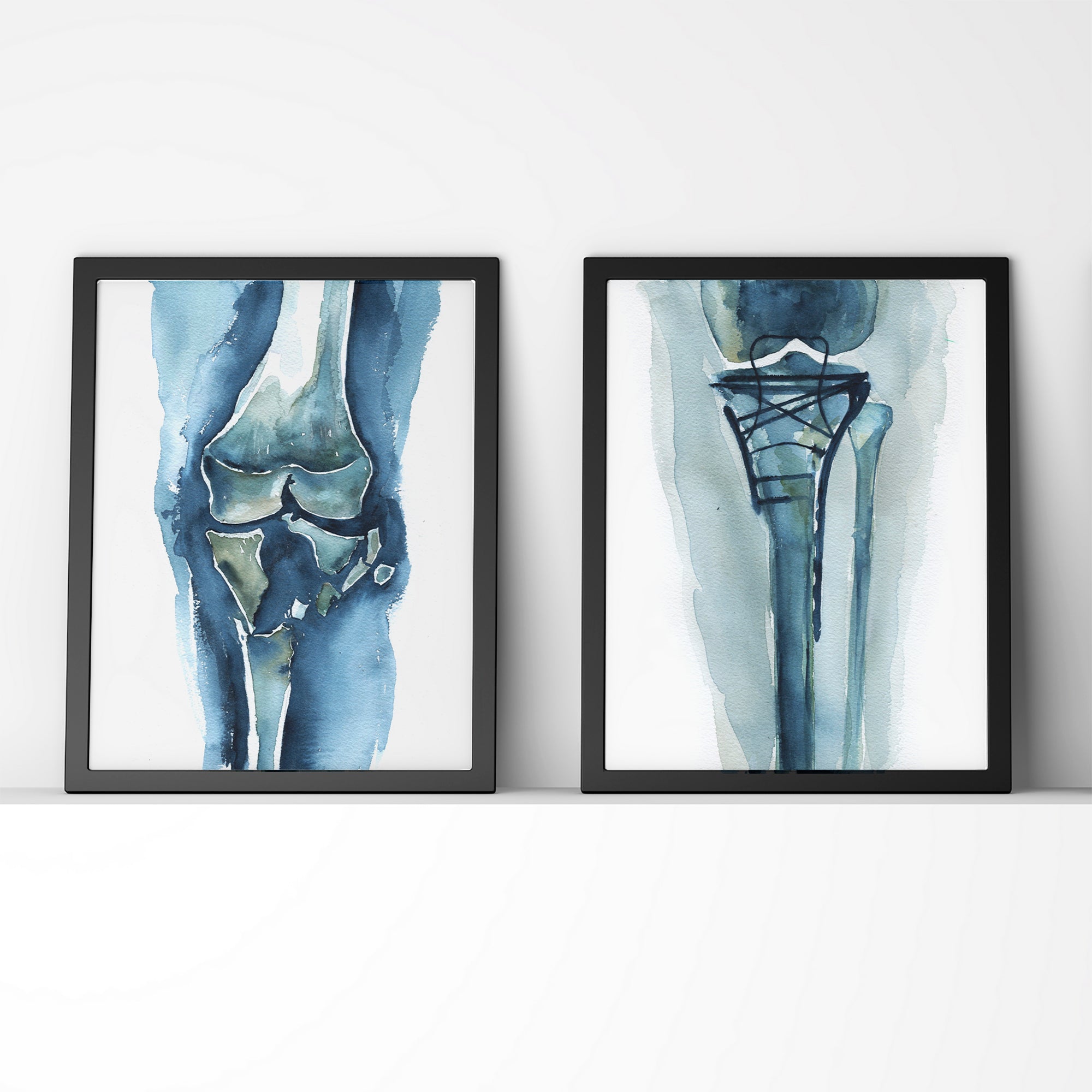The image depicts two framed watercolor paintings leaning against a white wall. Each painting is encased in a black frame, and the composition of the pieces brings attention to their medical theme. The painting on the left features an x-ray depiction of a broken knee, with various shades of blue watercolor depicting the leg's skin and bones. The bones are primarily dark blue with white accents, highlighting the fracture at the joint. The lines are somewhat abstract, not crisp or even, lending a unique artistic interpretation to the medical subject. The painting on the right portrays a broken leg, including visible leg bones and surgical repairs with wires, rods, and screws. This piece also predominantly uses blue watercolors, with the skin rendered in lighter blue tones and the bones in darker blue, accented with some darker grays. Both paintings feature lighter borders that blend into the off-white background of the image, emphasizing the framed artworks against the stark white wall.